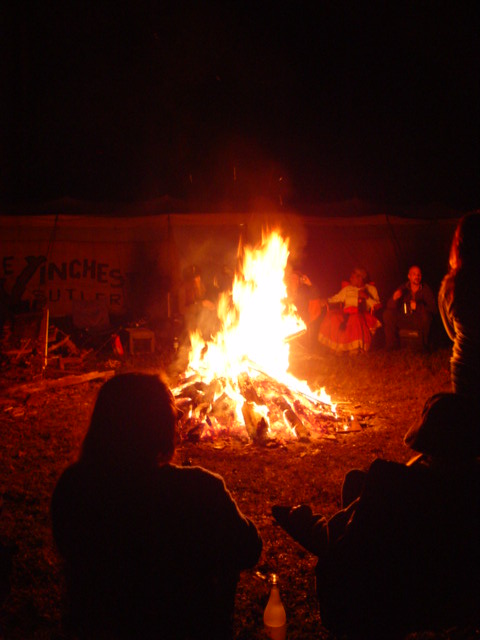The image depicts a nighttime bonfire, set against a dark, somewhat blurry background. At the center, a large, blazing campfire glows with bright orange and red hues, illuminating the scene. Several people are gathered around the fire, some sitting in chairs, others standing. In total, six individuals are visible. In the foreground, three people can be seen intently watching the flickering flames. Among the onlookers, there is a woman wearing a white shirt and a dress reminiscent of Native American attire, seated next to a bald man holding a cup. The background includes a wall with an indistinct sign that appears to read "Inches Butler," although the darkness and blurriness make it difficult to read clearly. The overall ambiance of the image captures a warm communal gathering amid the darkness of the night.